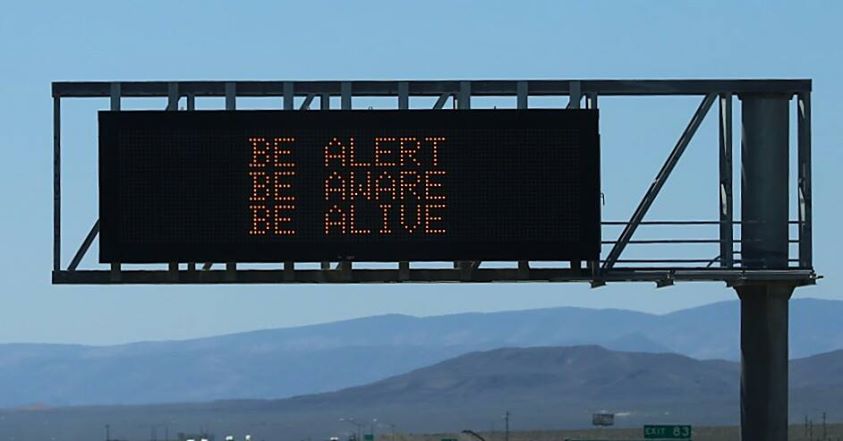In the image, there is a prominent digital street sign elevated high above the ground, supported by a robust, gray metal pole designed to hold various signs. The digital display on the sign features the message: "Be Alert, Be Aware, Be Alive," which is clearly visible from a distance. In the lower portion of the image, there is a secondary street sign indicating "Exit 83." The background depicts a slightly blurred horizon, suggesting the presence of heat, with tall mountains faintly visible in the distance.